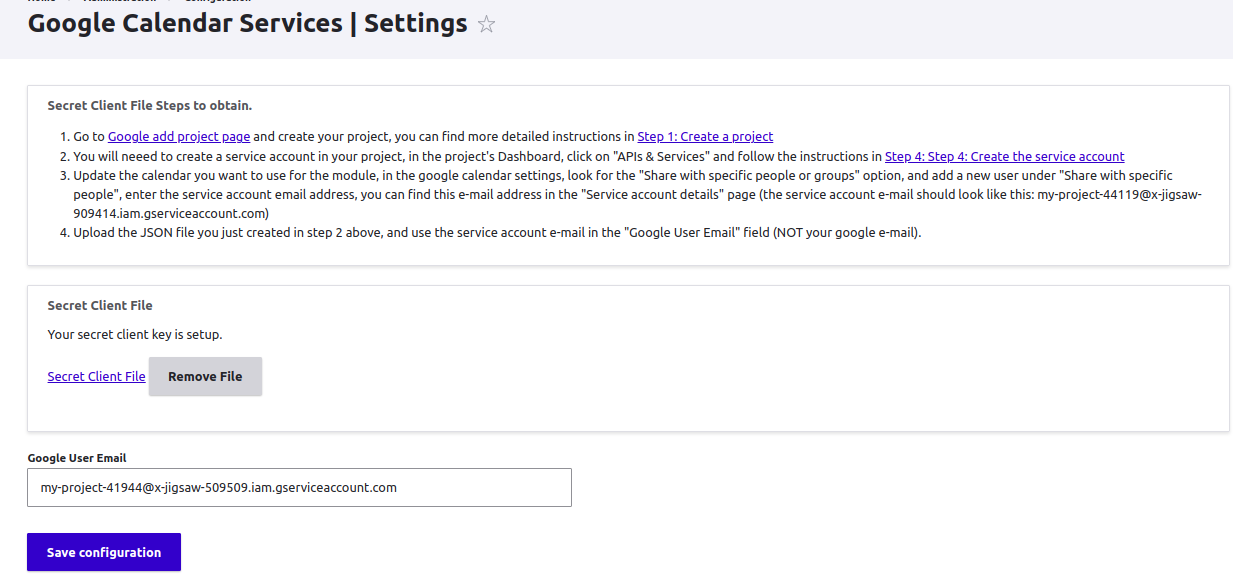The webpage features a header with a light blue or gray rectangle at the top, containing bold black text that reads "Google Calendar Services," followed by a vertical line, the word "Settings," and an unfilled star icon. Below this header, another section is titled "Secret Client File: Steps to Obtain."

The steps are listed numerically as follows:
1. Navigate to the Google Add Project page and create a new project. For detailed instructions, refer to "Step One: Create a Project."
2. Create a service account within your project. This is done via the Project Dashboard by clicking on "APIs and Services" and following the instructions provided in "Step Four: Create the Service Account."
3. In Google Calendar settings, update the calendar you intend to use for the module. Under "Share with specific people or groups," add a new user and input the service account email address found on the service account detail page. The service account email address should resemble "myproject44119@[domain].com."
4. Upload the JSON file created in Step Two, and use the service account email in the Google user email field, rather than your personal Google email.

At the bottom of the page, there is a light blue or gray rectangle labeled "Secret Client File." This section confirms that your secret client key is set up. Below it, there is a blue rectangle in the bottom left corner with "Google User Email" and "Save Configurations" displayed in white text.